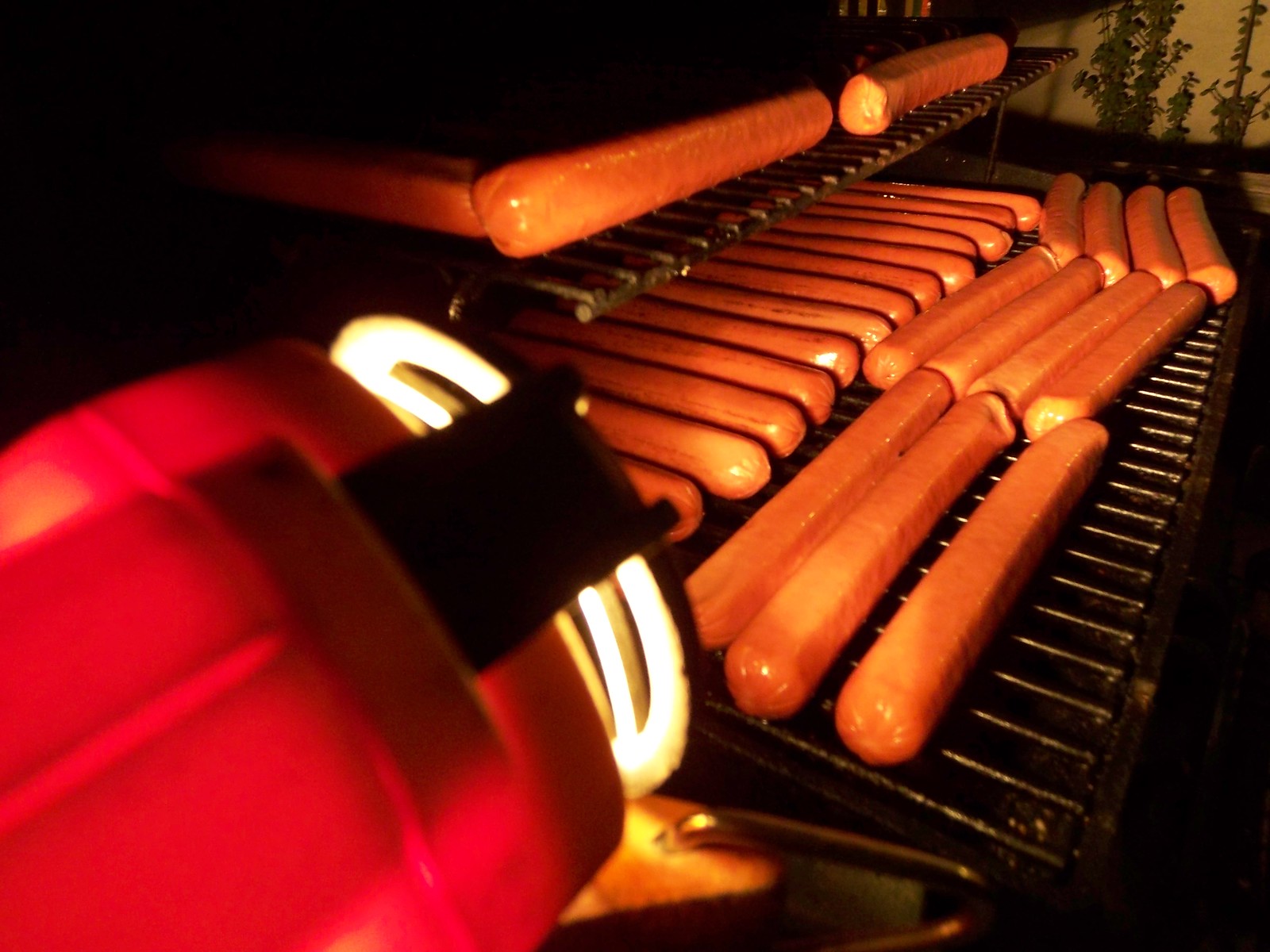The image depicts a nighttime scene of a grill heavily laden with hot dogs, covering nearly every inch of its surface. The main grill area features around two dozen hot dogs arranged both vertically and horizontally, with some showing clear signs of being nearly done, especially in the back row, while the front ones appear to have just started cooking. Additionally, there are three hot dogs positioned on the top warming rack at different angles. To the left, a red flashlight with a fluorescent light beam illuminates the scene, casting a bright glow on the hot dogs and contrasting with the overall darkness. The grill itself appears old and worn, suggesting frequent use. The background corners of the image remain obscured in shadows, indicating a lack of ambient light, befitting the nighttime setting.